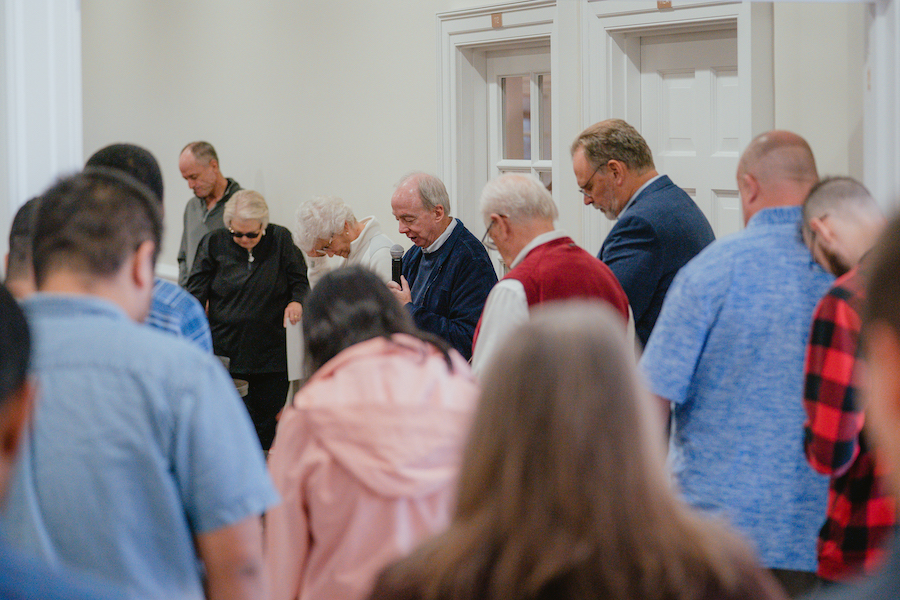The photograph depicts a prayer gathering in a spacious, white-walled room with visible windows and doors. Approximately 20 individuals are participating, forming a circle with several others standing behind them. At the center stands an elderly man, likely a minister, distinguished by his blue sweater over a white-collared shirt, gray hair, and a black microphone with a silver top. His head is slightly bowed, eyes possibly closed, immersing himself in the moment. The woman beside him has gray hair, glasses, and a drastically bowed head, while another woman in all black, including black sunglasses, stands next to her with her head also lowered. The room's casual attire ranges from red, blue, and pink, to checkered flannels, suggesting an informal yet solemn atmosphere. People closest to the camera have their backs to us and are slightly blurred, directing the focus towards the prayer circle and the minister at its center.